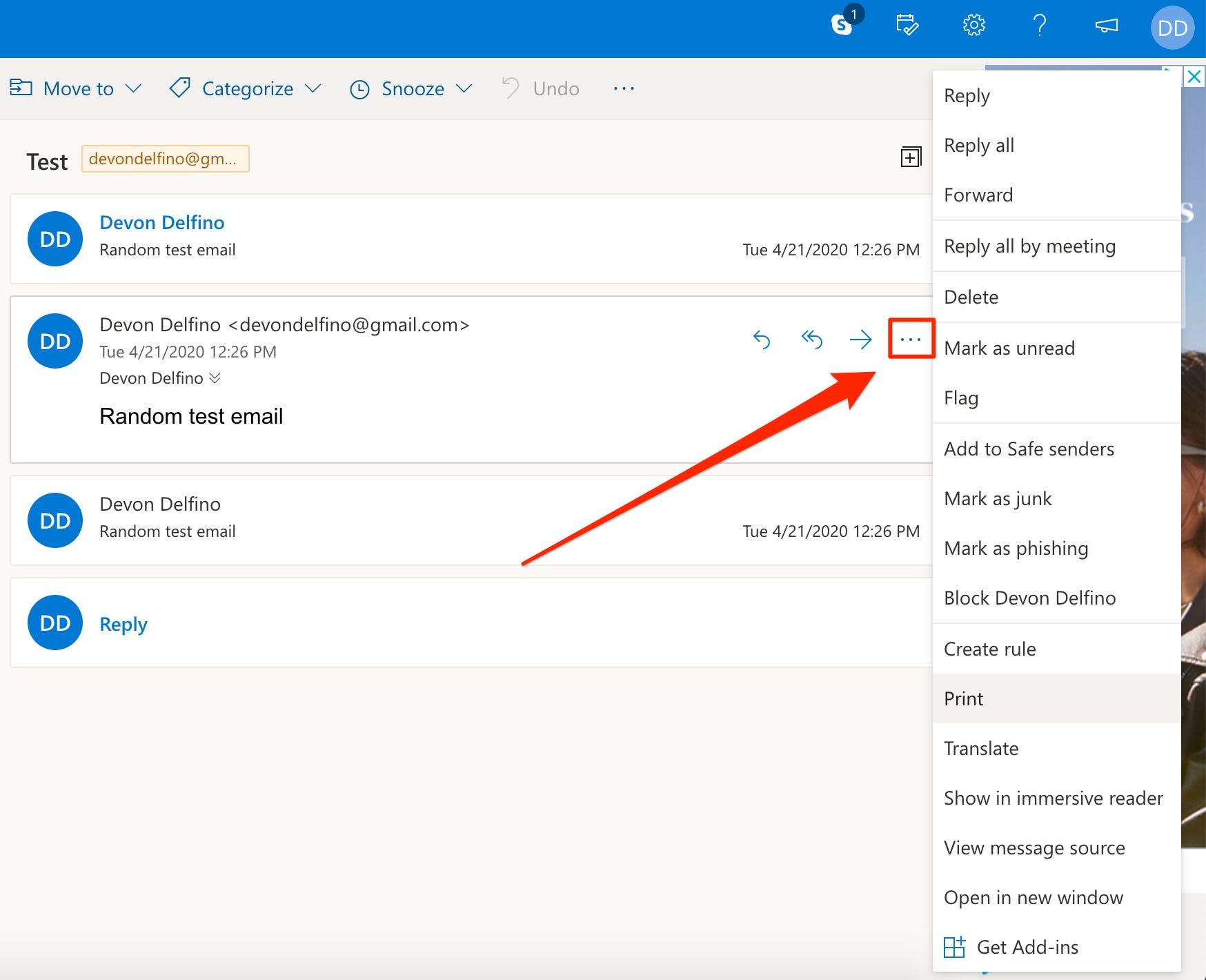The image depicts a section of an email interface with a colorful and detailed layout. At the top, part of the banner is blue and transitions into gray. The blue segment contains the options: "Move," "Categorize," and "Snooze," while the gray segment displays "Undo," followed by three blue circles.

On the right side, there's a prominent pop-up with various actions listed in black text, including: "Reply," "Reply All," "Forward," "Reply All by Me," "Delete," "Mark as Unread," "Flag," "Add to Safe Senders," "Mark as Junk," "Mark as Phishing," "Block," "Devon Devino," "Create Rule," "Print," "Translate," "Show in Immersive Reader," "Read Aloud," "Message," "Search," "Open in New Window," and "Get Add-ins."

To the left, in black text, appears the word "Test," situated above a brownish-colored box that reads "devondevino@gm..." The name "Devon Devino" appears in blue underneath the box. Below that, in black, is the text "Random test email," followed by a date and time: "Tuesday, 04/21/2012 11:26 PM."

Further down, various instances of the text "Devon Devino" and email address "devondevino@gmail.com" are displayed, along with the subject "Random test email." The date and time appear again as "Tuesday, 04/21/2020 11:26 PM." Navigational arrows, including two pointing backward and one pointing to the right, are highlighted with red boxes and arrows.

Lastly, at the bottom, the name "Devon Devino" appears again with "Random test email" and the date "Tuesday, 04/21/2020 12:26 PM" followed by a blue "Reply" option.